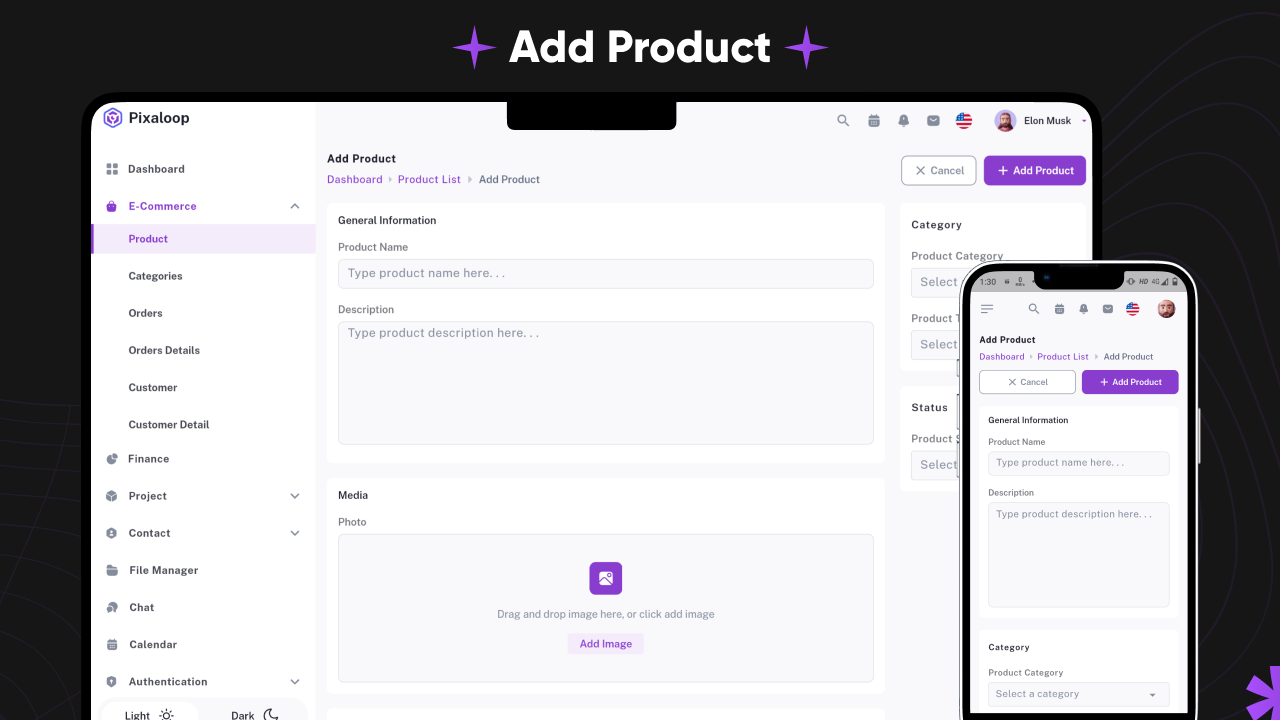Screenshot of an e-commerce product management page for a Pixaloop-based website. The interface enables users to add, organize, and manage products on their personal online stores. 

The top section prominently features an "Add Product" button, indicating the purpose of this page is to facilitate the addition of new products. 

The top-left corner displays "Pixaloop," the platform being used. Adjacent is an icon resembling a multi-sided shape with a purple circle at its center. 

A navigation sidebar on the left lists various options, with "Product" highlighted in purple, signaling the current selection. The navigation categories include:
- Dashboard
- E-commerce
- Categories
- Orders
- Order Details
- Customer
- Customer Detail
- Finance
- Project
- Contact
- File Manager
- Chat
- Calendar
- Authentication

A light and dark mode toggle is available at the bottom of the sidebar, accommodating users' preferences for interface appearance.

Below the "Add Product" header, a secondary navigation breakdown shows the following options: "Dashboard," "Product List," and "Add Product." The section beneath, titled "General Information," includes fields for "Product Name" and "Description," where users can input detailed information about the product they wish to add. 

Overall, the interface is designed to streamline the product addition process for online merchants using the Pixaloop platform.